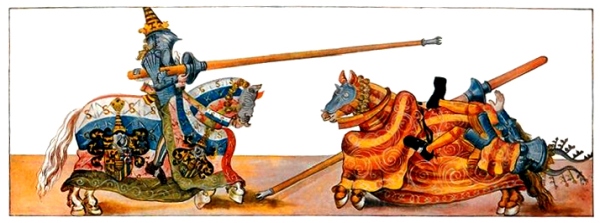This image depicts an old-timey, medieval illustration of a jousting scene between two knights on colorful, elaborately decorated horses. The horse on the left is vibrantly adorned in a striped cape of white, teal, orange, red, and green, with a white tail and a mostly white body. Its rider, clad in armor with a star-spangled, cone-shaped helmet, wields a jousting lance aimed at his opponent on the right. The knight on the right appears to have been unseated, falling from his horse, which sports gray, red, orange, and yellow stripes. The colors in the illustration are vivid, featuring blue, orange, red, green, brown, silver, black, and white, contributing to a warm, dynamic action shot. There is no text in the image. The characters have a somewhat fantastical appearance, with the knight on the left resembling a bird, adding to the enchanting, medieval atmosphere.